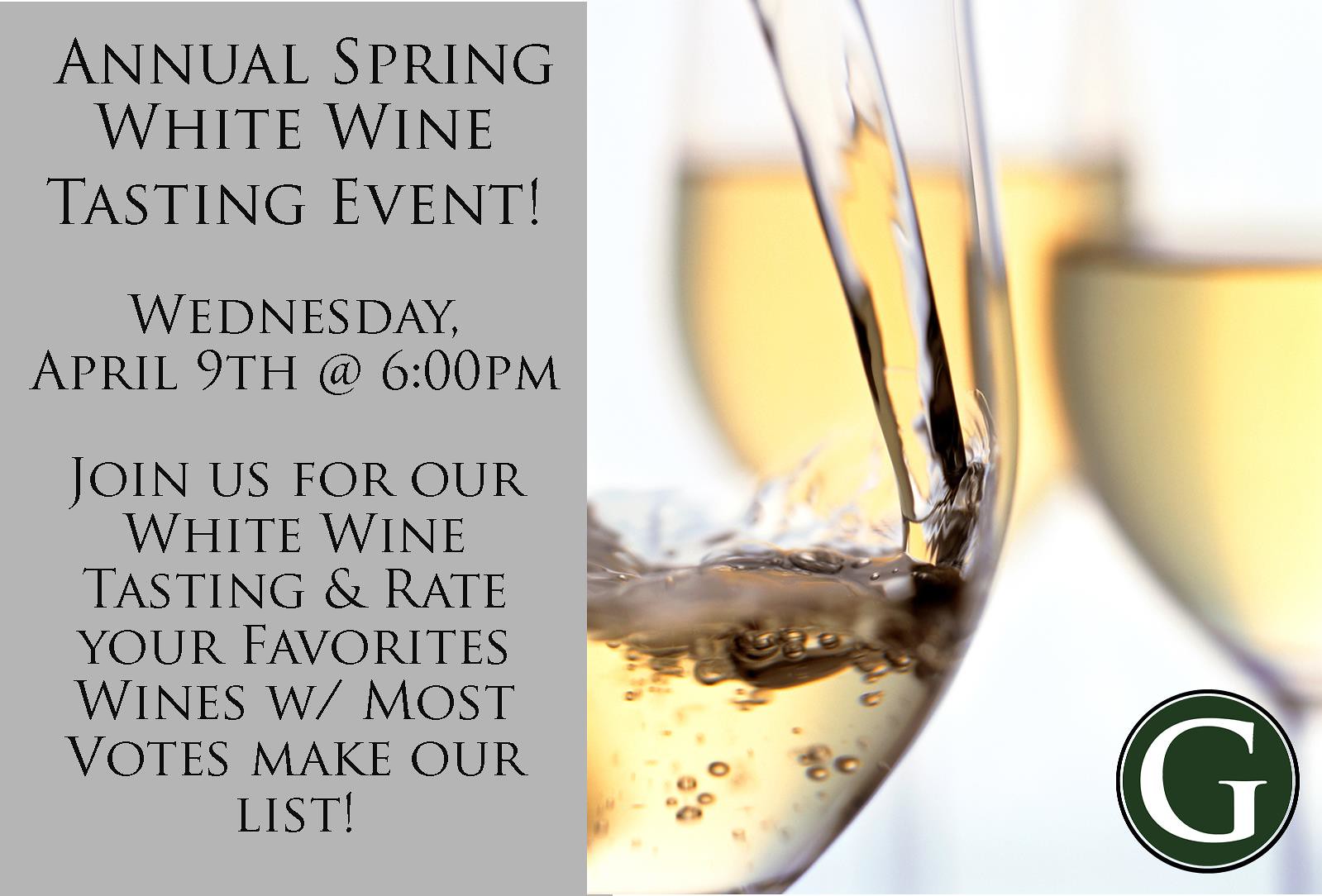Join us for our Annual Spring White Wine Tasting Event!

📅 **Wednesday, April 9th at 6 p.m.**

On the left side of the image, a light gray background features the details of the event in black text: "Annual Spring White Wine Tasting Event" at the top, followed by the date and time, and an invitation to join the tasting and rate your favorite wines. The text promises that the wines with the most votes will make it to their list.

On the right side, a close-up visual entices wine enthusiasts with a clear glass partially filled with a lightly tinted liquid, bubbling slightly at the lower level of the bowl. Behind the main glass, two additional glasses contain pale brown tinted wine. This setup highlights the variety of white wines up for tasting. At the bottom right corner, a green circle featuring a prominent white 'G' serves as a notable marker, likely representing the event's organizer or sponsor.